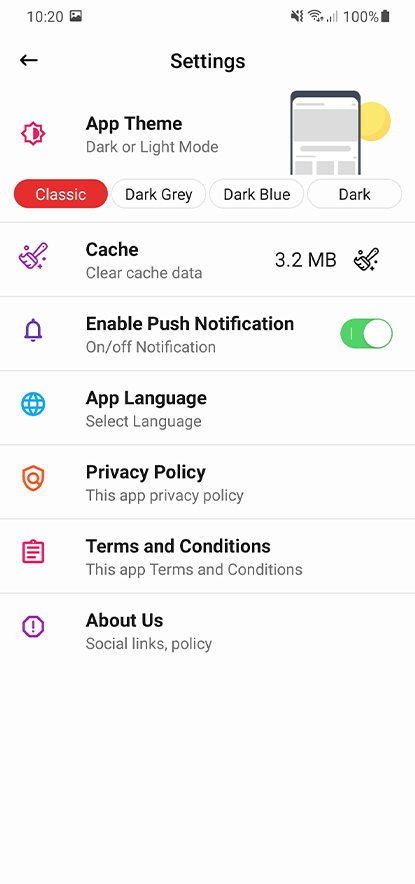**Caption**: 

This image showcases the settings page of a phone application. At the top edge of the screen, the upper left corner displays the time as 10:20 AM, while the upper right corner features a picture icon. Below the time, icons for no sound (vibrate mode), Wi-Fi signal bars, cell signal bars, and a 100% battery indicator can be seen.

Directly beneath this header, a left arrow appears on the left side, indicating a back navigation option. In the middle of the screen, "Settings" is prominently labeled. 

The settings are presented in a left-justified list, accompanied by a thin gray line separating each entry. The list is as follows:
1. **App Theme**: Options include Dark or Light Mode, Classic, Dark Gray, Blue, Dark Blue, and Dark. Currently, "Classic" is selected and highlighted in red, while the other options have black writing.
2. **Clear Cache**: Displays the cache data amount as 32.1 megabytes, with an option to clear it.
3. **Enable Push Notifications**: A toggle for push notifications is shown, which is currently switched on and indicated by a green color.
4. **App Language**: An option to select the app language, currently set to English.
5. **Privacy Policy**: Links to the app's privacy policy.
6. **Terms and Conditions**: Links to the app's terms and conditions.
7. **About**: Contains additional information about the app and its social links policies.

The colors visible in the image include red, pink, purple, blue, orange, green, yellow, white, black, and various shades of gray. The explanations for each setting are in gray text.